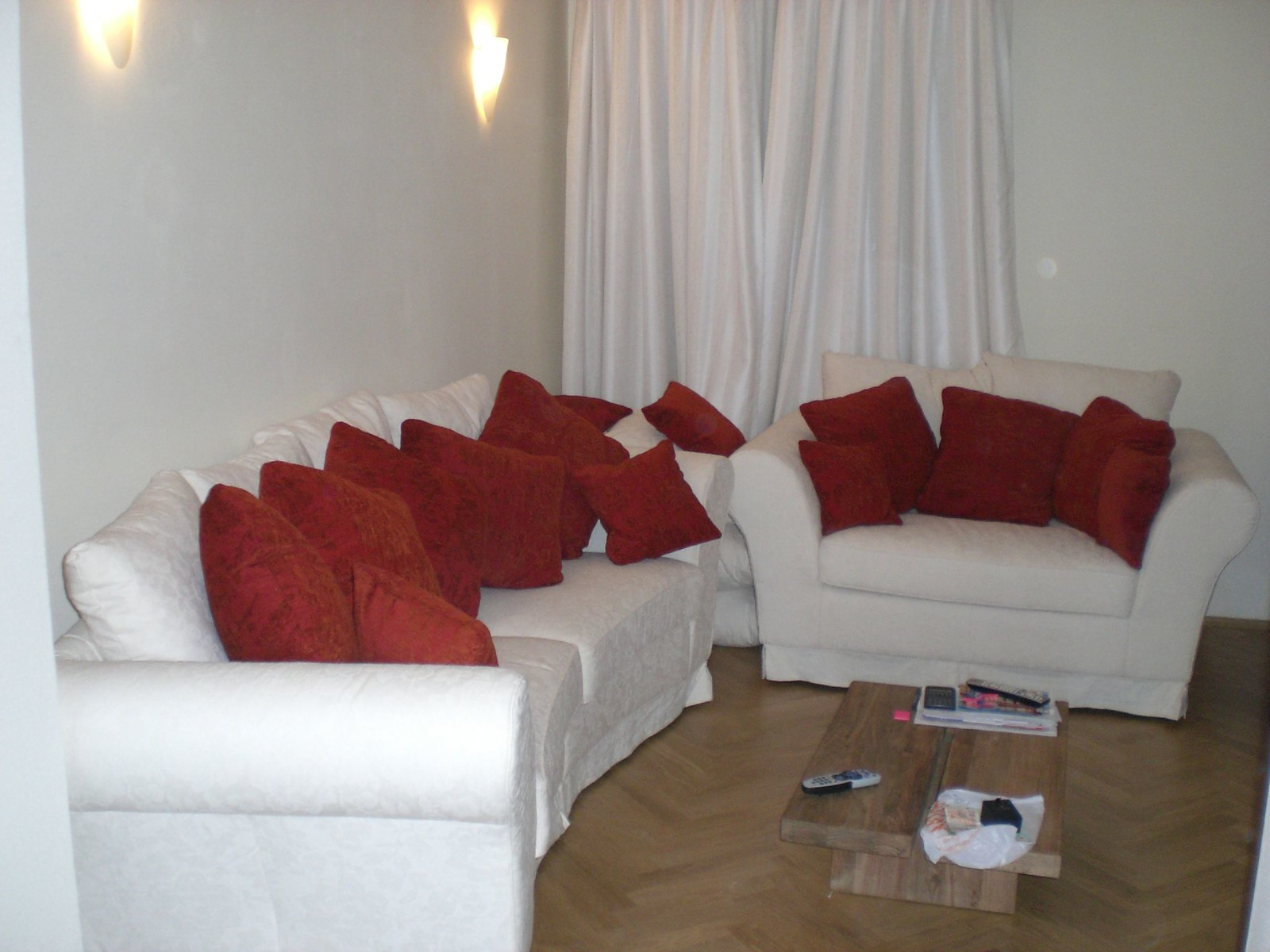This photograph showcases a well-lit, modern living room with a cohesive white and red color scheme. The room has plain white walls and is anchored by white curtains that span from the ceiling to the floor, covering a single window in the background. On the left wall, two stylish wall sconce lamps provide ambient lighting. The space features a light brown hardwood floor arranged in a chevron design, adding a touch of warmth to the room.

The seating in the living room includes a three-person couch and a two-person loveseat, both adorned with a mix of larger and smaller square red accent pillows. In the center of the seating arrangement is a short, rectangular wooden coffee table. On the coffee table, there are two remote controls, a stack of magazines, and a white plastic bag. The configuration and decor create an inviting and balanced atmosphere.